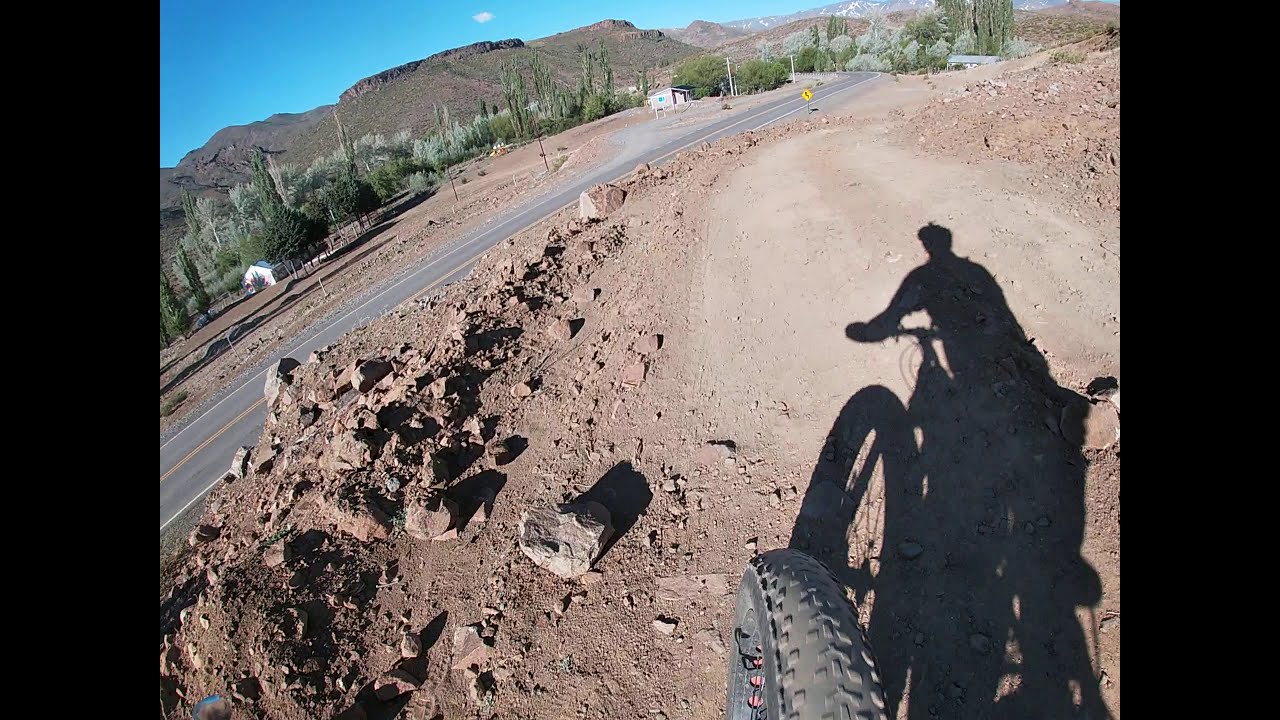The image captures a first-person perspective from a dirt bike rider as they navigate a curving, light-brown dirt trail in a desert landscape. The rider's shadow, cast by the late-day sun behind them, stretches prominently in front of the bike, showing the silhouette of the bike, the rider's gripping arm, helmeted head, and right foot. The front wheel of the dirt bike and the black edges of the photograph frame the scene. To the left of the trail lies a two-lane asphalt road with a yellow dividing line, flanked by cacti and other desert vegetation. Above the road, a small white shack is surrounded by trees, while another shack and distant plateau or mountain ridges are visible further down the center top. The sky is clear blue, enhancing the desert's arid, rugged beauty, reminiscent of the landscapes in Arizona or New Mexico.